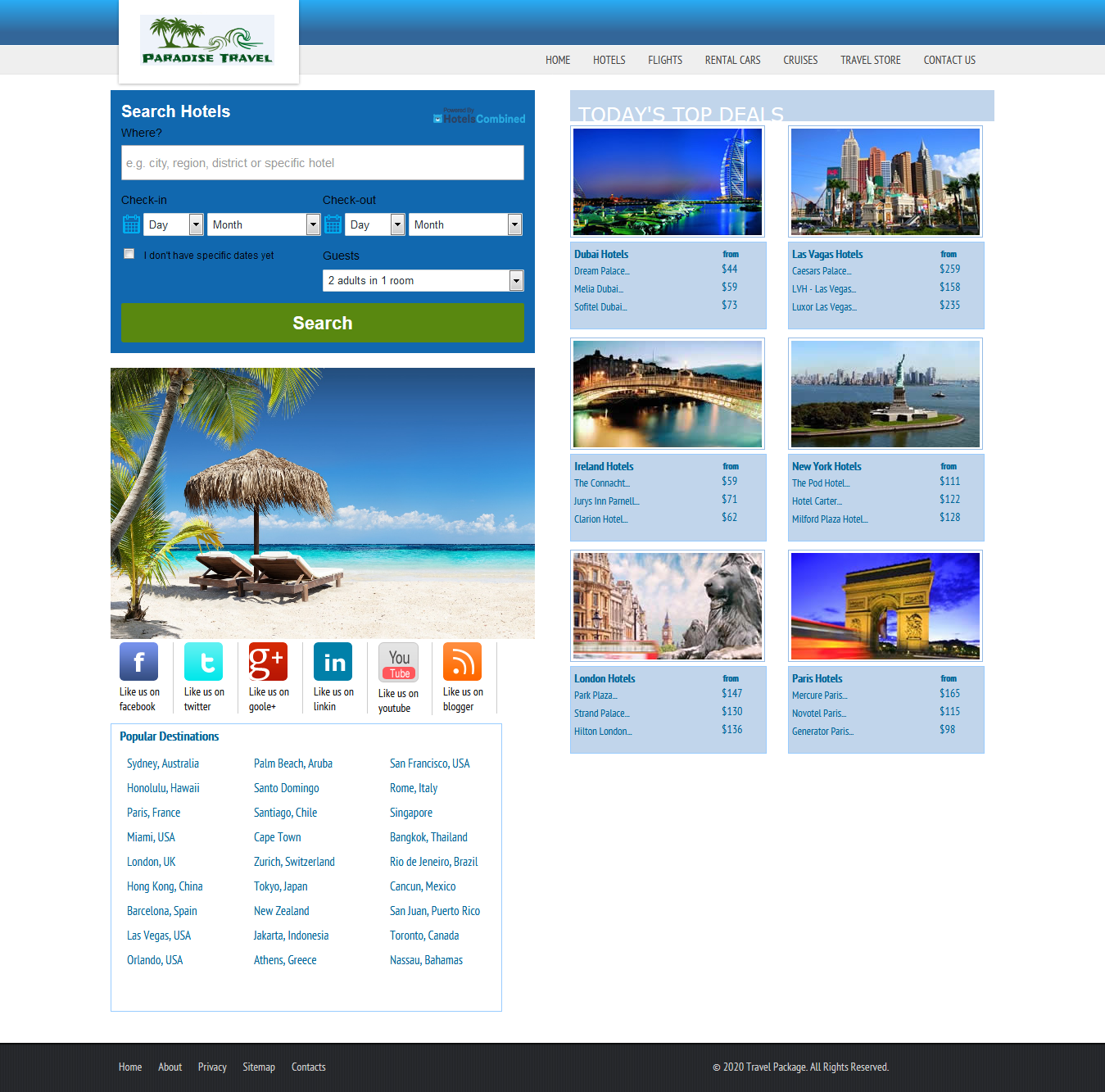The top of the image prominently displays "Paradise Travel" in vivid green letters against a scenic backdrop of lush, green palm trees. Below this header, there is a stylish blue box featuring a "Search Hotels" prompt. Just beneath the word "Where" is an open search box, allowing users to specify their destination. Adjacent to these fields, there are options to input check-in and check-out dates, culminating in a prominent, elongated green "Search" button.

The central portion of the image presents a picturesque illustration: an umbrella shading two lounge chairs placed on a pristine beach, with a swaying palm tree nearby, and the serene blue ocean stretching out in front of them. 

Below this idyllic scene, there's a row of social media icons enabling users to share or like the site on various platforms including Facebook, Twitter, Google, Instagram, and YouTube. 

To the right side of the image, a section labeled "Today's Top Deals" showcases six individual boxes featuring different travel destinations. The first box depicts a grand building illuminated against the night sky, with a body of water in the foreground, labeled as "Las Vegas Hotels." In the second row, a beautiful bridge arches over a calm expanse of water, followed by a representation of New York, marked by the iconic Statue of Liberty. The final row includes an image of a majestic lion standing near a tall building, and next to it, a quintessential red bus driving beside a recognizable towering structure, indicative of London.